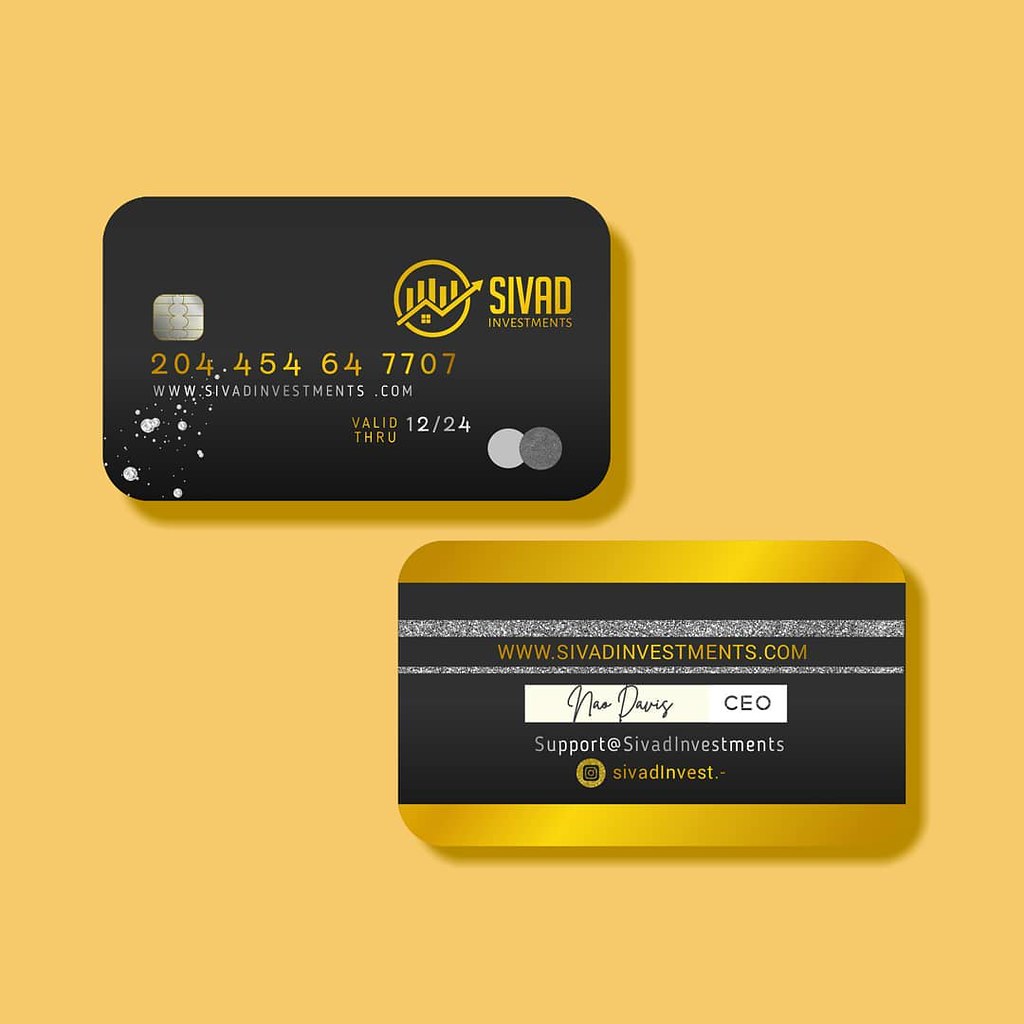This square image features a mustard yellow background and depicts both the front and back views of a credit card issued by CIVAD Investments. The front of the card, positioned towards the upper left, is predominantly black with rounded corners. At the top left, it features a silver chip reader. Below the chip, the card displays the number 204-454-647707 in gold text. Underneath the number, "www.civadinvestments.com" is printed in silver, while the card's expiry date, "valid through 12/24," appears in yellow and gray text. On the upper right side of the card, a gold circle logo with an upward arrow is displayed alongside the company name, "CIVAD Investments," in gold text. 

The back of the card is positioned towards the lower right and features a black rectangle in the middle with gold stripes on both the top and bottom edges. It prominently displays the name "CIVAD Investments" in gold text twice, with a space for a signature indicated by cursive writing next to the label "CEO." The back also includes the company website, "www.civadinvestments.com," in gold text, and an additional support contact, "support@civadinvestments.com," along with an Instagram logo. The card looks sophisticated with clear and detailed information, reflecting the branding of CIVAD Investments.